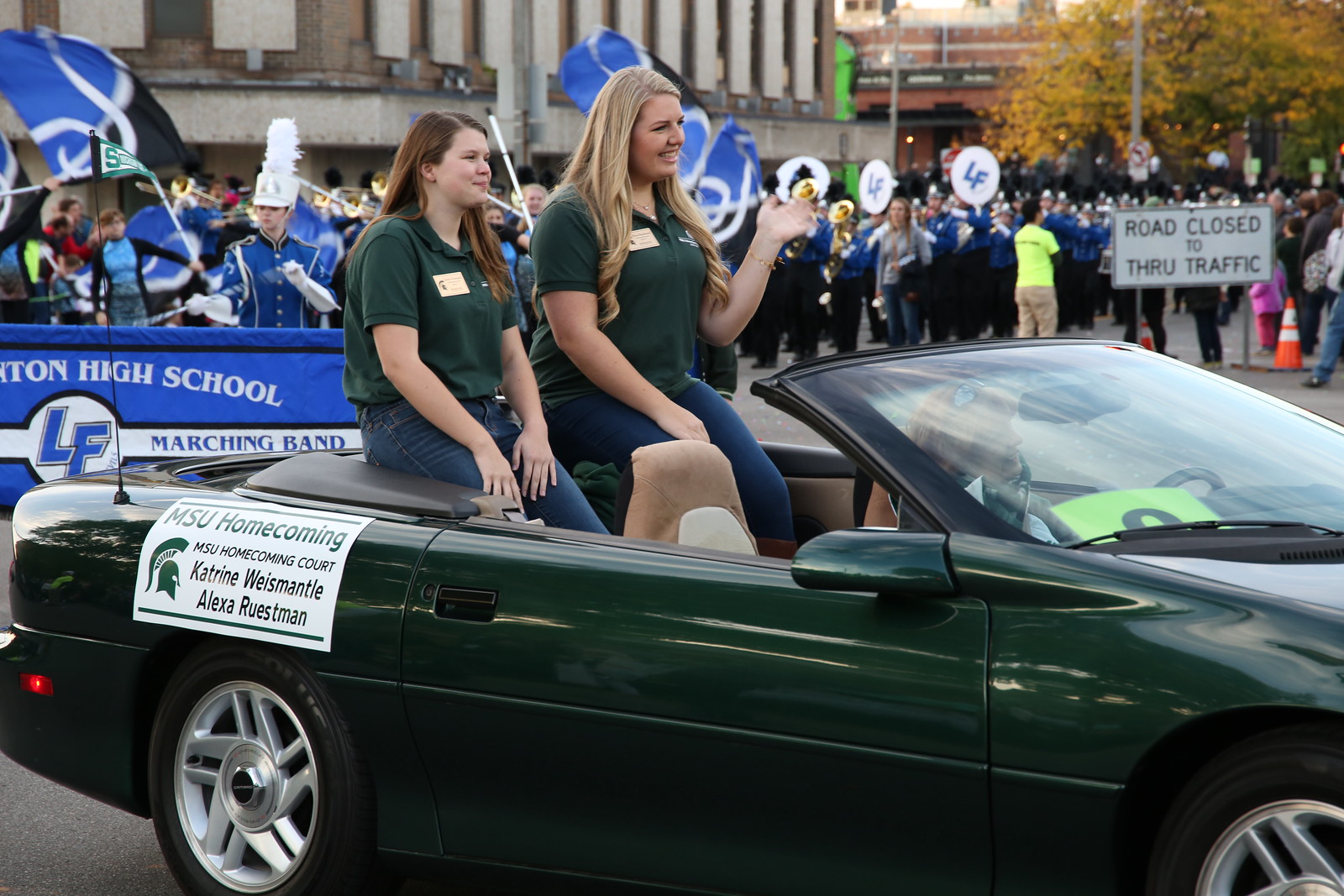The image captures a vibrant parade scene centered on a dark forest green convertible. The car, which lacks a roof, features two young women seated atop the back seats, wearing green polo shirts and dark blue jeans. The woman with blonde, curly hair waves to the crowd, while her companion, with straight brown hair, sits beside her. A sign on the car reads "MSU Homecoming Court: Katrine Westmantle and Alexa Roosman." In the background, a lively crowd cheers, separated from the parade by a "Road Closed to Through Traffic" sign. Directly behind the convertible, members of a high school marching band, dressed in blue uniforms, carry a partially visible blue banner with the words "high school" and "marching band." Among the band members, a figure holding a pole can be seen, adding to the festive atmosphere. The backdrop includes a building and several trees, enhancing the depth and context of this bustling parade scene.